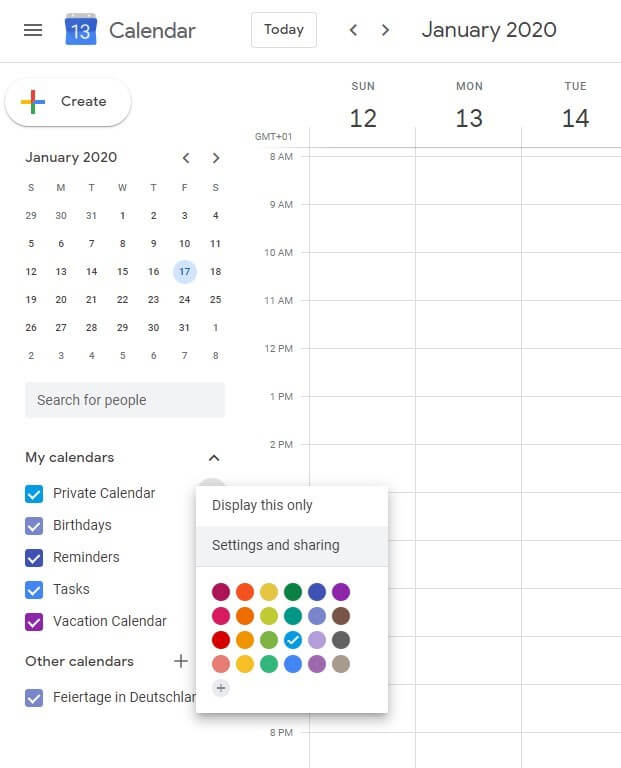The image appears to be a screenshot of a calendar app on a mobile device, likely a cell phone or tablet. At the top of the application, there is a menu section accessible via an icon on the top left. The current date is clearly indicated as the 13th, with a "Today" button highlighting this date. To the right of the "Today" button, the text "January 2020" is displayed, accompanied by navigational arrows that allow users to switch between months.

The calendar interface seems to be from Google Calendar, identifiable by the distinct "+" sign on the "Create" button. The main display features a monthly view of January and a weekly view showing specific dates such as Sunday the 12th, Monday the 13th, and Tuesday the 14th. Time slots are listed along the left side of the weekly planner, ranging from 8 a.m. to 2 p.m., although the lower times are partially obscured. Each day displayed in the week view includes a segmented layout allowing users to input events or tasks.

Additional interface elements include a full monthly calendar where the 17th is notably highlighted. A search bar for finding people is also present. On the right-hand side, there's a "My Calendars" section that allows users to manage various calendar categories such as "Private Calendar," "Birthdays," "Reminders," "Tasks," and "Vacation Calendar," each identifiable by checkboxes in different colors. There is also an option to add other calendars. On the left side, a pop-up window is visible, offering color customization for various calendar elements.